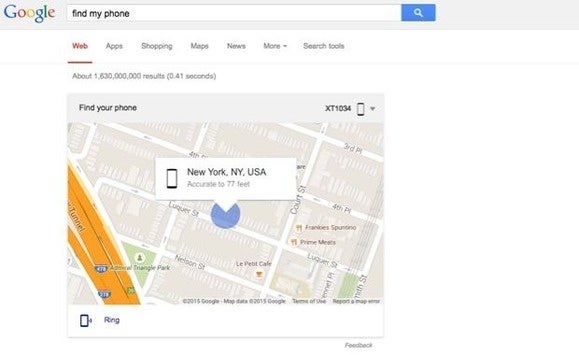A screenshot shows the Google "Find My Phone" feature in action. The interface displays a drop-down menu with options including web, apps, shopping, maps, news, and more. The search result, completed in 0.41 seconds, highlights the location of the phone model XT1034, with an accuracy of 77 feet. The map pinpoints the phone's location on Luquer Street in New York, NY, USA. The screen includes various options like "Ring" and "Feedback," with additional details such as "Maps data 2015" and terms of use links. The overall layout showcases the efficiency and detail provided by Google's search and mapping technology in 2015.